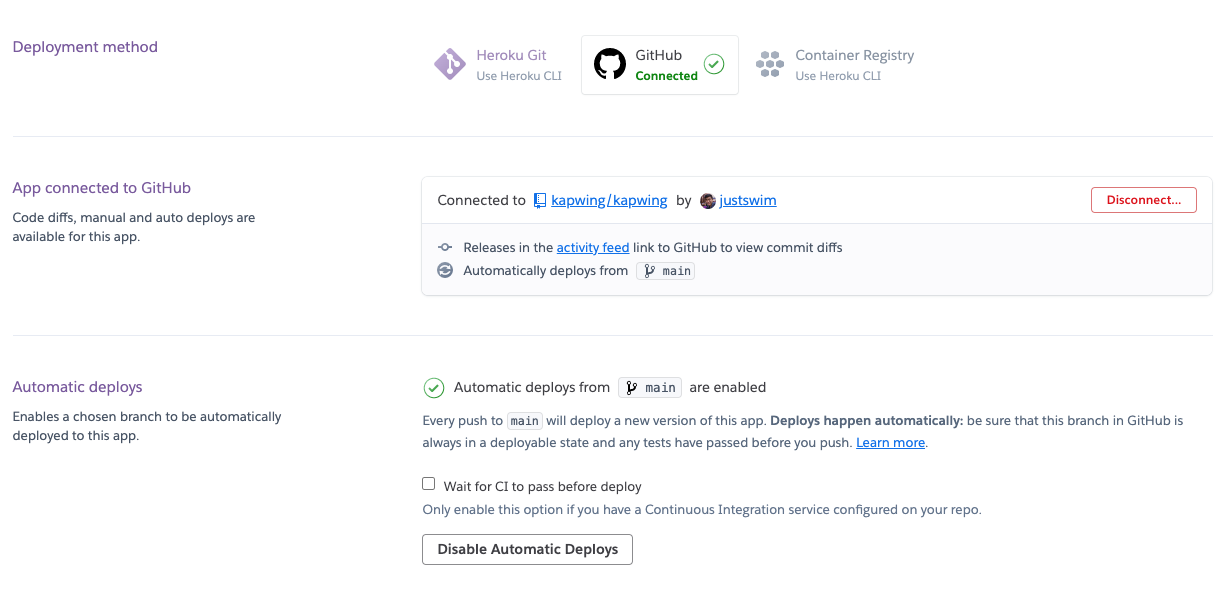Caption: 

The image displays a detailed view of a deployment dashboard for a web application, highlighting various deployment methods and configurations. The left panel shows that the application is connected to GitHub, listing options like Heroku, Git, GitHub, Connected, and Container Registry. The middle section indicates that the app is linked to the "capwing/capwing" repository by Jetswim, featuring a small profile picture and a highlighted "Releases" section in the activity feed.

The interface further outlines different deployment options, mentioning code diffs and the availability of both manual and automatic displays for the app. A notable feature is the "Automatic Deploys," which ensures that a chosen branch is automatically deployed to the app. There is an emphasis on connecting to the main branch, with the message that every push to the main branch will trigger a new deployment version. Users are advised to verify that the main branch is deployment-ready and all tests have passed before pushing changes.

Additionally, the interface suggests enabling the option to wait for Continuous Integration (CI) to pass before deployment. This is recommended only if a continuous integration service is configured. The option to disable automatic deploys is also present for further customization.

Overall, the image provides a clear and comprehensive overview of the deployment setup, emphasizing the importance of automated processes and CI in ensuring smooth and reliable updates to the application.